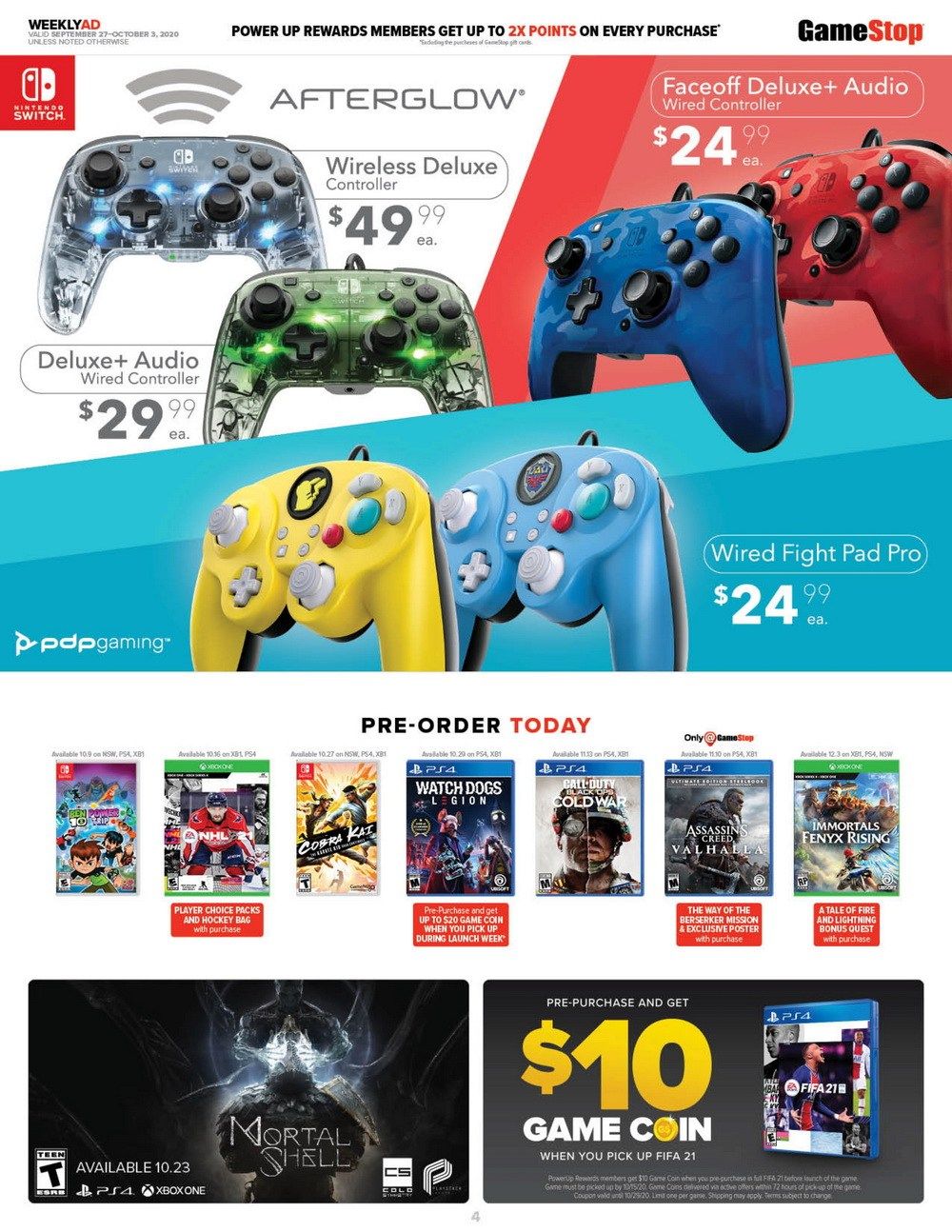A screenshot of a Nintendo-themed website showcases an array of game controllers, prominently featuring Afterglow models. Displayed prices range from $24.99 to $149.99. The site highlights a pre-order for the game "Mortal Shell," available starting October 23. The background features dynamic hues of blue, red, and white, adding a vibrant touch to the website's design. Various other games are also visible in the background, enhancing the gaming ambiance.